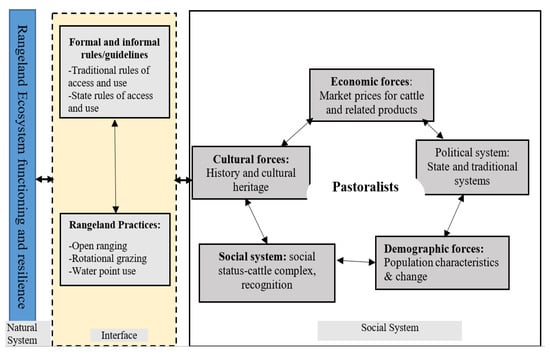The diagram illustrates the interrelations within a rangeland ecosystem, focusing on its functioning and resilience. On the left side, there's a beige rectangle bordered by a dotted line, divided into two sections: the top box labeled "Formal and Informal Rules and Guidelines" and the bottom box titled "Rangeland Practices," which details open ranging, rotational grazing, and water point use. 

To the right of this, there is a large central square with a black border containing five internal rectangles, each connected by two-way arrows. At the top center, the box labeled "Economic Forces" discusses market prices for cattle and related products. Below it, the central box emphasizes "Pastoralists." The left middle box, labeled "Cultural Forces," delves into history and cultural heritage. Below this, the "Social System" box addresses social status and cattle complex recognition. On the right side, the middle box titled "Political System" covers state and traditional systems. The bottom right box, "Demographic Forces," highlights population characteristics and changes.

Each of these rectangles is interconnected with two-way arrows, signifying dynamic interactions among economic, cultural, political, demographic, and social factors influencing the rangeland ecosystem.